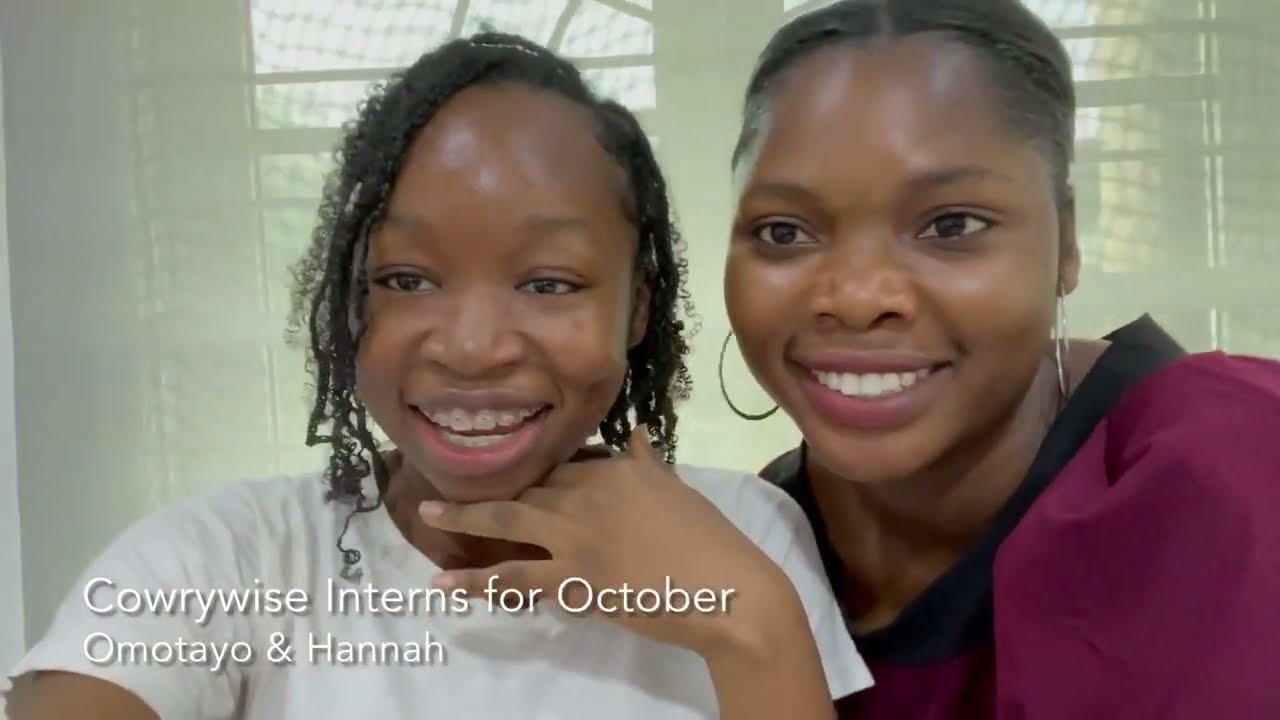The image features two African-American females who appear to be a mother and daughter. The younger woman, positioned on the left, is a teenager with tight spirals of hair falling down the sides of her face and braces on her teeth, adding a youthful charm to her big, bright smile. She wears a white short-sleeved T-shirt and has her left hand thoughtfully resting under her chin, with her right arm extended forward. The older woman, standing slightly over her left shoulder on the right side of the image, is elegantly dressed in a maroon or burgundy blouse with a black neckline. Her hair is slicked back with subtle braids highlighting it, and she accessorizes with silver-hooped earrings and matching pink-tinted lipstick. She has wide-set brown eyes and a broad smile showcasing her nice white teeth. Behind them is a window with drapes. The text overlay at the bottom reads "Cowrie Wise Interns for October, Omotayo and Hannah," suggesting a professional setting for this image.